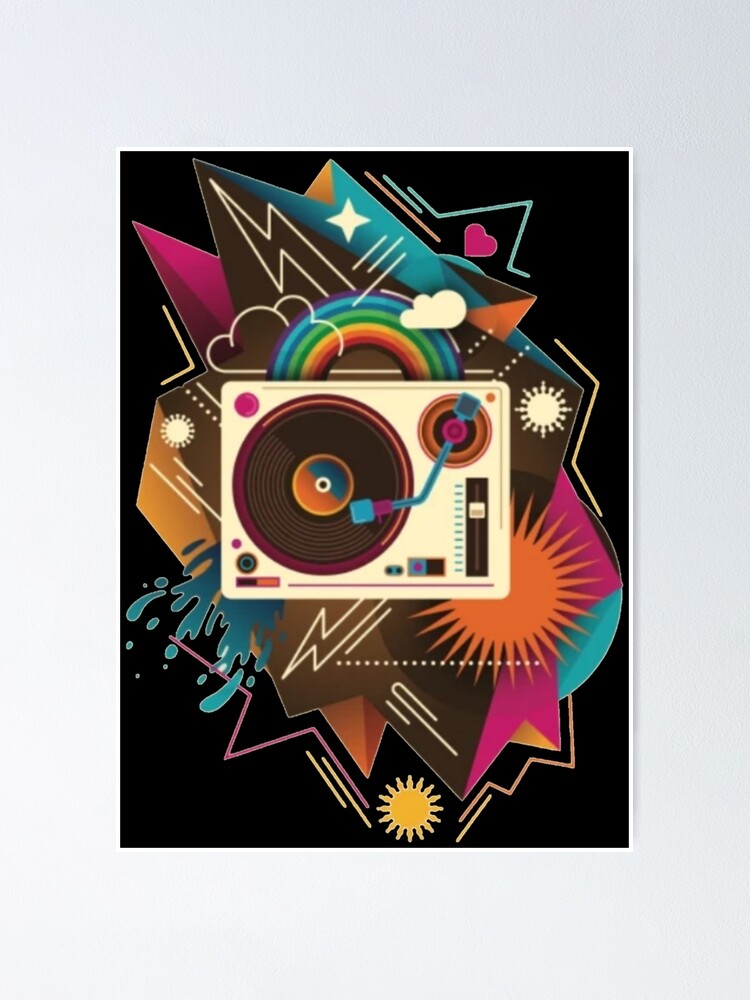The image features a retro, abstract 2D style poster set against a black background. Central to the composition is a beige, rectangular briefcase-like object resembling a turntable or phonograph, complete with a rainbow handle. At the center of this object lies a dark brown LP record, accented with blue and pink. The turntable's stylus is depicted in blue and pink, poised on the record. Surrounding the turntable are various vibrant elements including two sunbursts—one yellow and one orange—alongside a pink heart. The scene is peppered with an intricate mix of abstract shapes: white cloud outlines, a rainbow, starbursts, and a prominent lightning bolt. The overall color palette includes blue, pink, orange, and yellow, bringing dynamic energy to the retro-themed artwork.